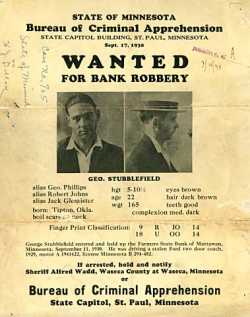The image depicts an aged, sepia-toned wanted poster from the State of Minnesota, dated September 17, 1938, issued by the Bureau of Criminal Apprehension, located at the State Capitol Building in St. Paul, Minnesota. The poster seeks the apprehension of a bank robbery suspect referred to as G.O. Stubblefield, with various aliases including Allison G.O. Phillips, Robert Jones, and Jack Gallagher. The poster features two black-and-white photographs of the suspect: one frontal portrait and a side profile, where the suspect is dressed in a black blazer, white collared shirt, and a straw bolero hat in the side profile image. Detailed physical descriptors include age 22, height 5'10", weight 165 pounds, with brown eyes, dark brown short hair, good teeth, and a medium dark complexion. The poster emphasizes that if arrested, authorities should hold the suspect and notify Sheriff Alfred Wadd of Wasilla County, Minnesota, or the Bureau of Criminal Apprehension in St. Paul, Minnesota. The document features several illegible handwritten notes along the margins.